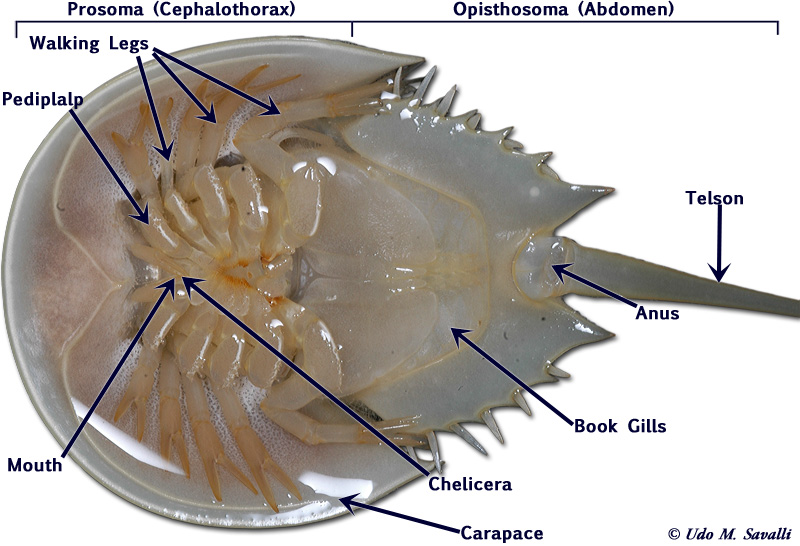This image is an anatomical photograph, likely intended for a textbook, depicting the underside of a sea creature that resembles a stingray. The sea creature, which has a circular body tapering to a pointy tail, is predominantly grayish-blue with brown highlights and appears to have a slimy texture. The image is meticulously labeled in black writing with black arrows pointing to various anatomical parts.

The creature's body is divided into two main sections: the prosoma (cephalothorax) and the opisthosoma (abdomen). The prosoma houses the walking legs, pedipalps, mouth, carapace, and chelicerae. The opisthosoma includes the book gills, anus, and telson. Sharp spikes or tentacles are visible along its backside, which stop just before the tail. Labels for all these parts are clearly denoted, making this image a comprehensive diagram of the creature's anatomy.